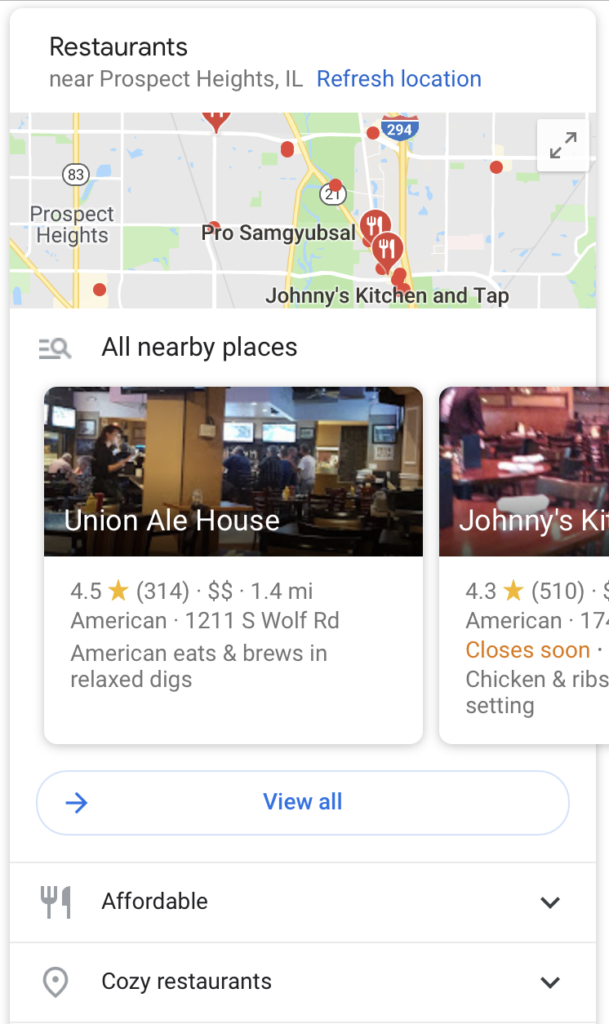This screenshot from a website showcasing local restaurants, likely sourced from Google Maps, visually represents a search query for dining options in the user's vicinity. The user specifically appears to be located near Prospect Heights, IL. The search results highlight several restaurant choices, each accompanied by ratings and distance from the user's current location. For instance, the Union Ale House is featured with an impressive 4.5-star rating based on 314 reviews and is situated 1.4 miles away. Another option, Johnny's Kitchen and Tap, has garnered a 4.3-star rating from 510 reviews and is noted to be closing soon. Additional filtering options are visible, allowing the user to refine their search further by categories such as affordability and coziness. A small map displaying red markers pinpoints the precise locations of these restaurants, providing an easy visual reference for proximity.